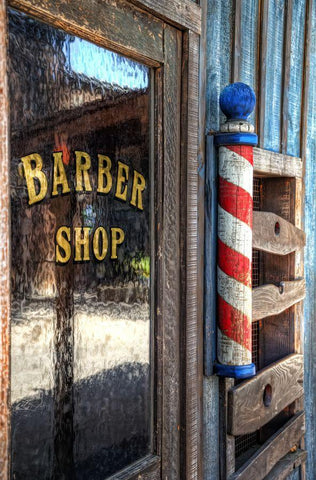This image captures a close-up of an old-style barber shop that has been boarded up, exuding a nostalgic charm. The door, located on the left, is framed in old wood with a glass window. Across this window, in large, gold uppercase letters outlined in black, the words "BARBER SHOP" are prominently displayed. Adjacent to the door, on the right, stands a classic barber pole, showcasing the iconic red and white candy-cane stripes with a blue finial on top and a blue base at the bottom. Beside the barber pole is a boarded-up window, covered with large wooden slats nailed across it. The exterior of the building is painted a sea blue color, suggesting a once-vibrant establishment. Through the glass window, one can faintly see the reflection of the street and another building across from it, adding depth to the scene.